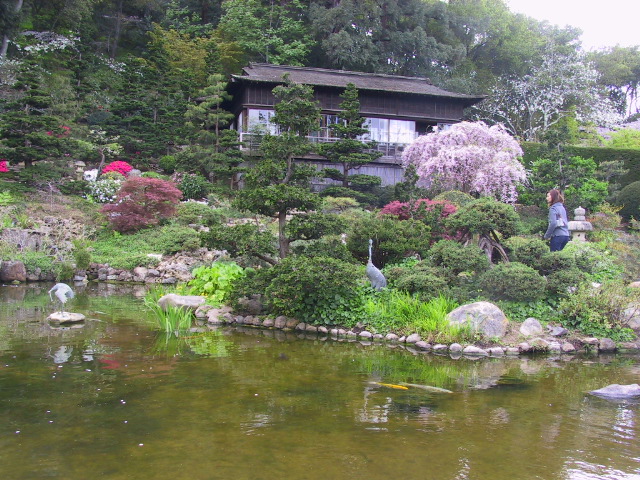This highly detailed color photograph captures a serene hillside scene, featuring a charming house with a pagoda-style roof surrounded by a lush forest. The house, viewed from the side and built into the hills, is flanked by numerous windows reflecting the verdant backdrop of tightly packed trees. In front of the house lies a tranquil, almost circular pond edged with stones and greenery, home to colorful koi fish – including a striking goldfish and a yellow one. A graceful willow tree with its cascading branches and a variety of vibrant bushes, some in bright and dark pink hues, enhance the rich landscaping around the pond. Amongst the bushes and stones stands a woman, the only human in the photograph, with brown hair, dressed in navy blue pants and a long-sleeve top or jacket. Her side is turned to the camera as she walks towards the house. Additionally, a gray crane bird is visible in the lush landscape, adding to the picturesque nature of this peaceful garden scene.